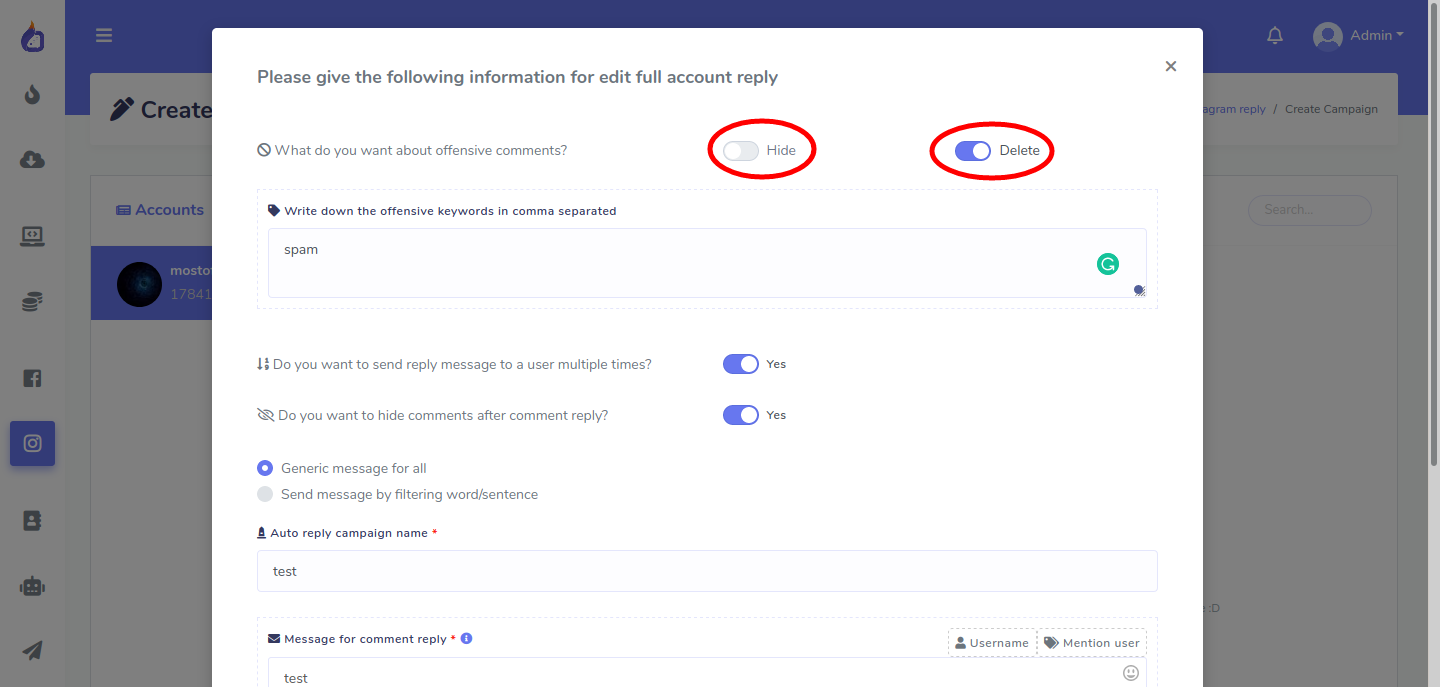This screenshot captures an interface of a computer application. In the background, there's a dark blue bar at the top of the screen, accompanied by a gray, slightly blurred background featuring additional options that appear dimmed and not in active focus.

Dominating the screen's foreground is a large white dialog box, occupying over two-thirds of the visible area. At the top of this box is the title: "Please give the following information for full edit account reply," alongside an 'X' button on the right side for closing the menu.

Within this dialog box, several options and fields are available for interaction:

1. **Offensive Comments Management**:
   - **Question**: "What do we want to do about offensive comments?" 
   - **Options**:
     - **Hide choice**: Represented by a slide button, currently deselected.
     - **Delete choice**: Another slide button, positioned to the right and highlighted, indicating it is selected.

2. **Keywords Entry**:
   - Label: "Write down the offensive keywords, separated by commas."
   - A rectangular text entry box containing the word "spam."

3. **Reply Message Settings**:
   - **Option**: "Send a reply message to the user multiple times."
     - A slide switch highlighted to 'Yes.'
   - **Option**: "Do you want to hide comments after a comment reply?"
     - A slide switch in the 'Yes' position.

4. **Message Sending Preferences**:
   - Two radio buttons are present:
     - **Selected**: "Generic messages for all."
     - **Not Selected**: "Send messages by filtering word/sentence."

5. **Auto Reply Campaign Details**:
   - Label: "Auto reply campaign name."
   - Text entry box populated with the word "test."
  
6. **Message or Comment Reply**:
   - Label: "Message or comment reply."
   - Attachments options include: User name and mention user.
   - Text entry box also containing the word "test."

This detailed menu appears to be tailored for managing and customizing responses within the application, especially focusing on managing offensive content and setting up automated replies.